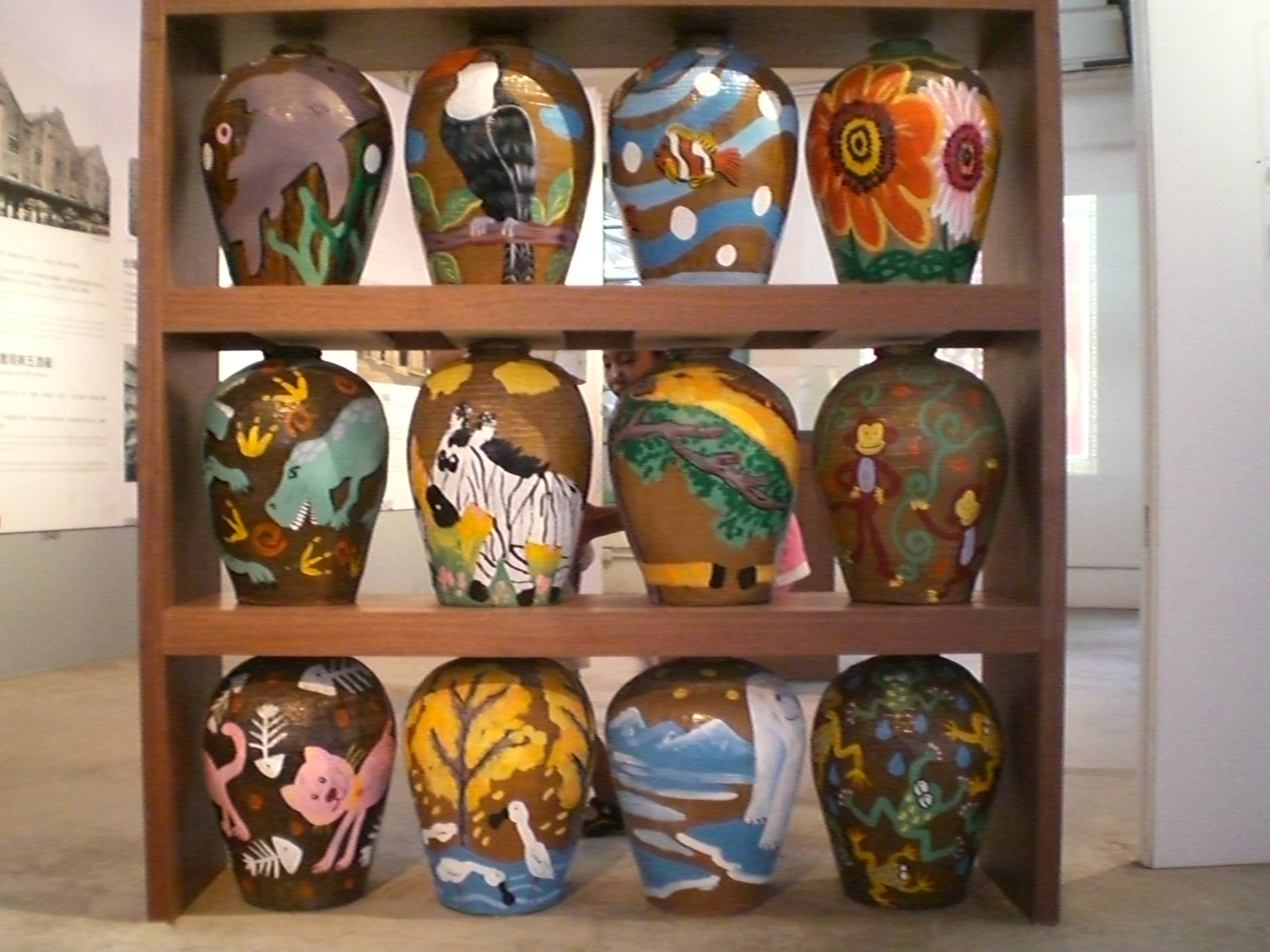This photograph was taken indoors, possibly in a museum or a pottery class display, showcasing a brown wooden shelf with three layers, each adorned with four large, colorful vases, making a total of 12 vases. The shelf is positioned on a carpeted floor in a spacious room, with sunlight streaming through a window in the background. To the left of the shelf, there's an illustration of a structure with some text underneath it, though it's unreadable from this distance.

The vases boast a vibrant array of colors, including blues, reds, pinks, browns, greens, yellows, and purples, each hand-painted with intricate designs predominantly featuring outdoor animal scenes. On the top shelf, one vase displays a shark in an underwater scene, another shows a black parrot with an orange beak, a third illustrates a fish swimming amidst water bubbles, and the fourth features big orange and pink flowers.

The middle shelf includes a vase with green dinosaurs and their footprints, another with a striped zebra in motion, a third showing a giraffe eating leaves from a tree, and the fourth with playful monkeys swinging in a jungle setting.

The bottom shelf consists of a vase with pink cats and skeletal fish, one with ducks or geese swimming in a pond against a backdrop of trees, another depicting a polar bear on ice with snowy mountains in the background, and the last vase showing frogs jumping from lily pad to lily pad with detailed water drops painted around.

Each vase vividly captures the artistic expressions of their creators, exhibiting a blend of animal themes and nature scenes.